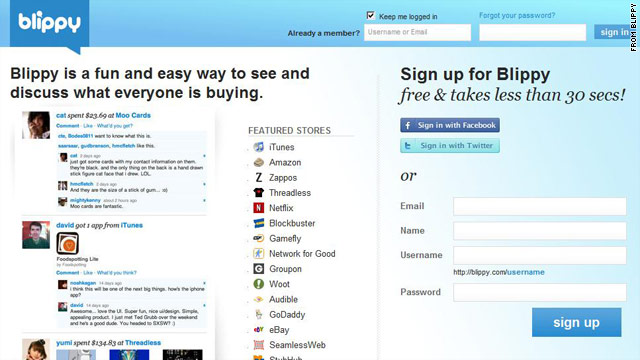The image depicts a website with a background in white and pastel blue hues. In the upper left corner, within a blue rectangular shape, the word "Blippi" is prominently displayed in white text. The word "Blippi" is spelled B-L-I-P-P-Y. Below "Blippi," on the left side, there's a phrase written in black text that reads: "Blippi is a fun and easy way to discuss what everyone is buying."

Directly beneath this description, several profile pictures are showcased, each accompanied by comments written in either blue or black text. 

In the middle right section of the image, there is a column labeled "Featured Stores." Under this heading, names of several stores, including iTunes, Amazon, Zappos, and Threadless, are listed.

On the far right side of the image, a sign-up form for Blippi is featured. The top of this form has a caption that reads: "Sign up for Blippi free and takes less than 30 seconds."